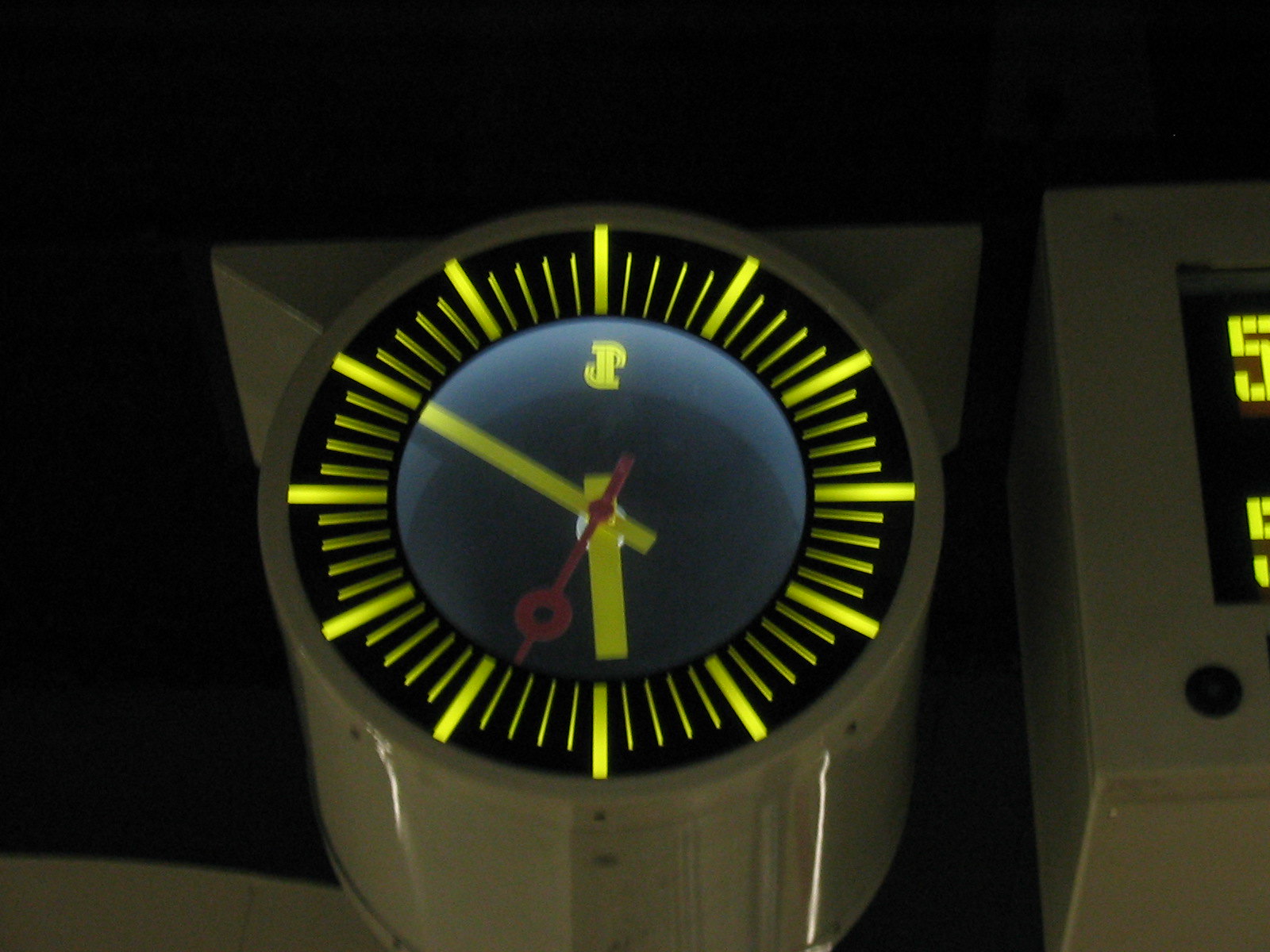The image depicts a close-up view of a white or medium gray plastic mechanical device, resembling a clock or meter, set against a solid black background. The apparatus is primarily circular with a distinct clock-like face showing hour, minute, and second hands illuminated in bright yellow and fluorescent green, with the second hand in red. Despite lacking numerical digits, the clock face displays larger lines for hours and smaller lines for minutes. A decorative 'P' logo is centered on the clock face, possibly indicating branding. Adjacent to this clock-like device, there is another piece of equipment, partly visible, that appears to be a rectangular or square digital unit. This secondary device displays the number '5' twice, and it shares the same color scheme, reinforcing a cohesive design. The overall appearance and setup suggest the equipment might have nautical applications.